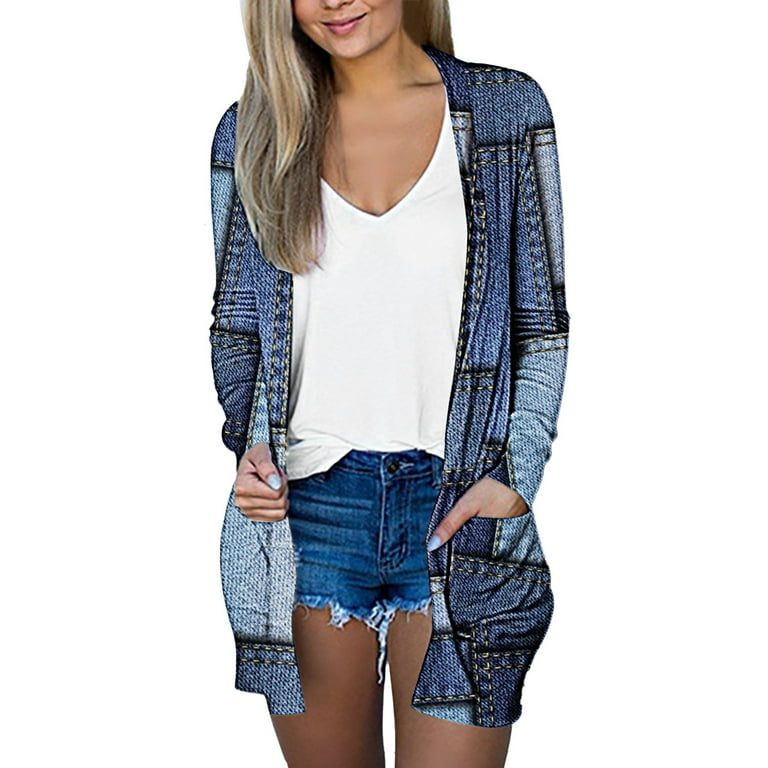The photograph showcases a female model from her nose down to her thighs, set against a plain white background. She has long, straight blonde hair and is wearing pink lipstick. Dressed in a white v-neck t-shirt, mostly tucked in with the front out on both sides, she pairs it with very short, dark blue, frayed blue jean shorts. Over this, she wears a distinctive patterned sweater, adorned with various shades of blue squares and intersected with black lines and yellow stitching, resembling jean material but potentially silk-screened. The sweater extends three to four inches below the shorts, creating a layered look. Completing her outfit, she sports light blue fingernail polish. The focus is clearly on her and her clothing, reminiscent of images commonly used by clothing retailers.